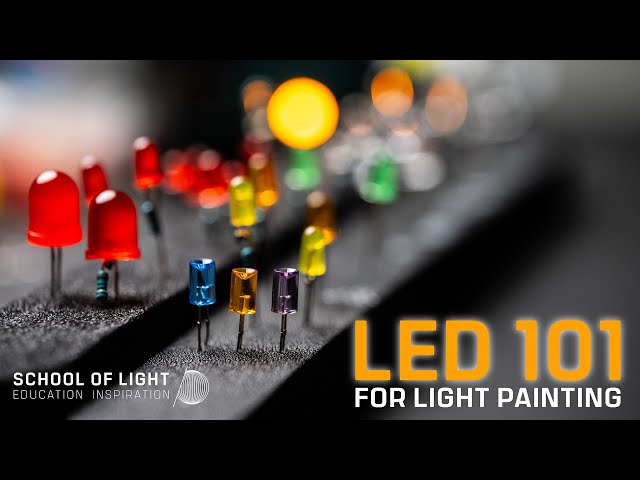The photograph depicts a collection of LED lights embedded in long, black strips resembling pushpins. The image is predominantly out of focus, except for a few lights on the left side, which are sharply detailed. On the black boards, LEDs of various shapes and colors are arranged. Notably, there are two larger, dome-shaped red lights on the left, followed by smaller, cylindrical lights in blue, yellow, and dark blue. The bottom left corner of the image features the text "School of Light Education Inspiration" in white, and the bottom right corner displays "LED 101" in orange letters, with "For Light Painting" underneath in white. The boards appear to be at different heights, and most of the lights in the background are blurred, creating a soft depth of field.